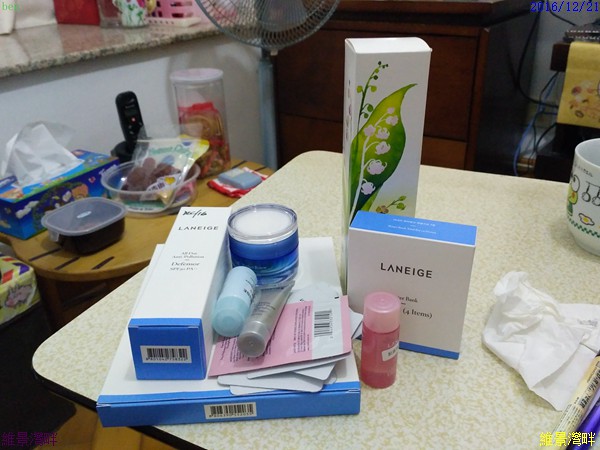In this image, a cluttered room is depicted with numerous items scattered across various surfaces. In the foreground, a small, foldable Formica table holds a disorganized pile of personal grooming products, including lotion and possibly concealer, which appear to have just been taken out of a bag. A tissue and a white mug with green and yellow accents, featuring an illustration of an egg, sit beside the grooming products. 

To the left, a child-sized table contributes to the disarray, holding a box of tissues, a plastic Rubbermaid container of unknown contents, a bowl with cookies inside a bag, and an old-fashioned cordless telephone. A standing fan is positioned adjacent to this small table.

Behind the fan, a marble counter top supports a pink basket and a red box. Further in the background, a stand, likely holding a TV, adds to the overall cluttered appearance of the room.